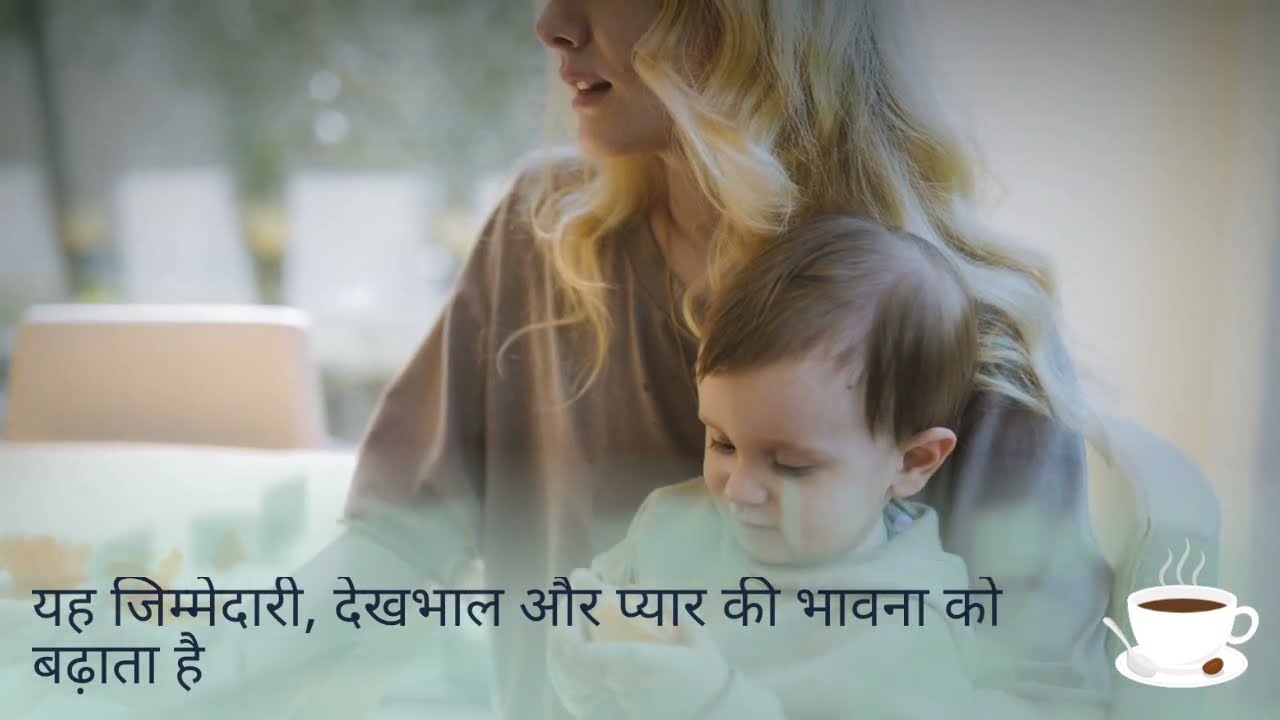This photograph features a woman with long, curled blonde hair, visible only from her nose down. She is wearing a brown long-sleeve shirt and has a very young child, around one year old, sitting on her lap. The child holds an object in his hands, gazing down at it intently, while the woman looks in a different direction. The setting appears to be indoors, likely within a house or building, with some indistinct white objects visible in the background. Along the bottom of the image, there's text written in a foreign language, possibly from the Middle East. In the lower right corner, a cartoony graphic of a steaming coffee cup on a saucer is present, adding a whimsical touch. The image’s color palette includes shades of white, brown, black, green, and yellow, suggesting a brightly lit scene, possibly taken during the day.